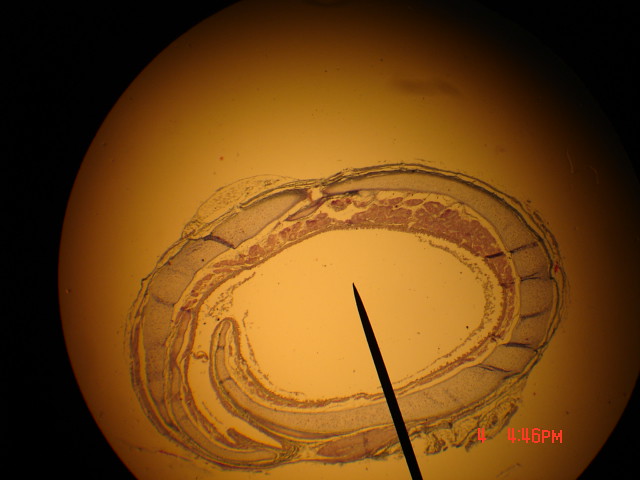The image portrays a medical or scientific slide being displayed, possibly as part of a presentation. At the center of the photo is an egg-like or oval-shaped object with varying shades of tan and orange. At the lighter center of the object, a darker pointer or needle, shaded in black, appears to be either injecting into or pointing towards the center from the bottom right of the image. The background is completely black, adding stark contrast to the illuminated object and the pointer.

The timestamp, "4:46 p.m.," is displayed in red font in the bottom right corner. The oval shape has a gradient, lightening towards the center and darkening towards the outer edge, indicating that it might be under a specific lighting condition or projection. The overall clarity of the image is quite high, highlighting the intricate details of the pointer and the object it interacts with.